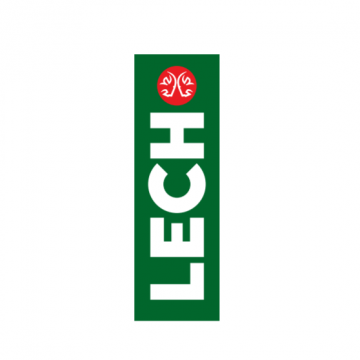The image features a business logo set against a blank white background. Central to the composition is a vertically oriented, dark green rectangular block, taller than it is wide. From a 90-degree counterclockwise rotated perspective, bold white capital letters spell out "LECH" (L-E-C-H) along the length of the rectangle. Positioned above the rectangle, there is a red circle containing a white design that resembles two goat heads colliding, with their horns meeting at two distinct points. The striking contrast of green, red, and white elements against the plain background makes this logo visually prominent and easy to identify.